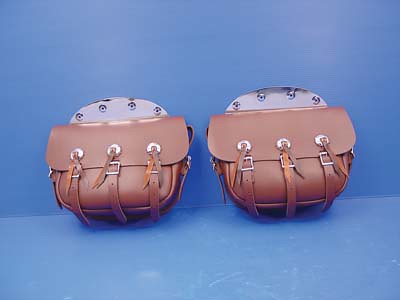This color photograph showcases two identical brown leather saddlebags propped side by side against a seamless blue backdrop that extends from the vertical surface to the horizontal base, creating a professional studio setting. Each saddlebag, crafted from light brown leather, features three front straps secured with brass buckles that bind the top flap to the body of the bag. The top part of each bag includes a distinctive semi-circular grayish metal component adorned with four circular metal rivets or buttons arranged in an arc. The bags are slightly rounded at the bottom, sitting full and structured, and lack visible hand straps. The lighting from above casts subtle shadows, accentuating the smooth leather surfaces and the detailed embellishments.